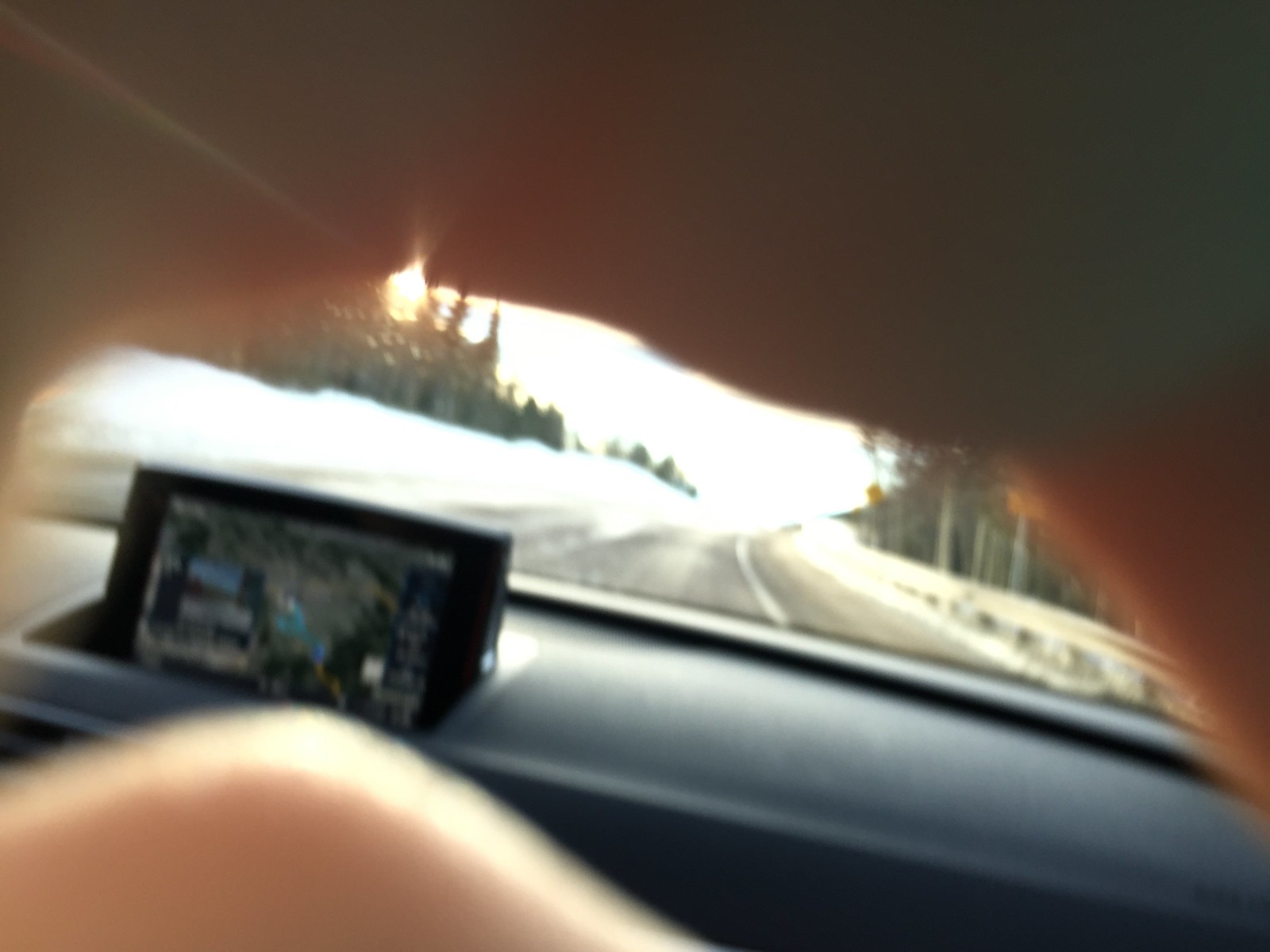This outdoor color photograph, slightly wider than it is tall, appears to have been taken from inside a car, looking through the front windshield. The image is partially obscured by a hand, which casts a flesh-colored blur across the top and right side, with additional obstruction from what might be a finger in the bottom left corner. Despite these obstructions, the scene outside the windshield reveals a snowy landscape featuring a road flanked by trees on both sides. The dark dashboard of the car is visible, with a small pop-up screen on the left side displaying an indistinct image.